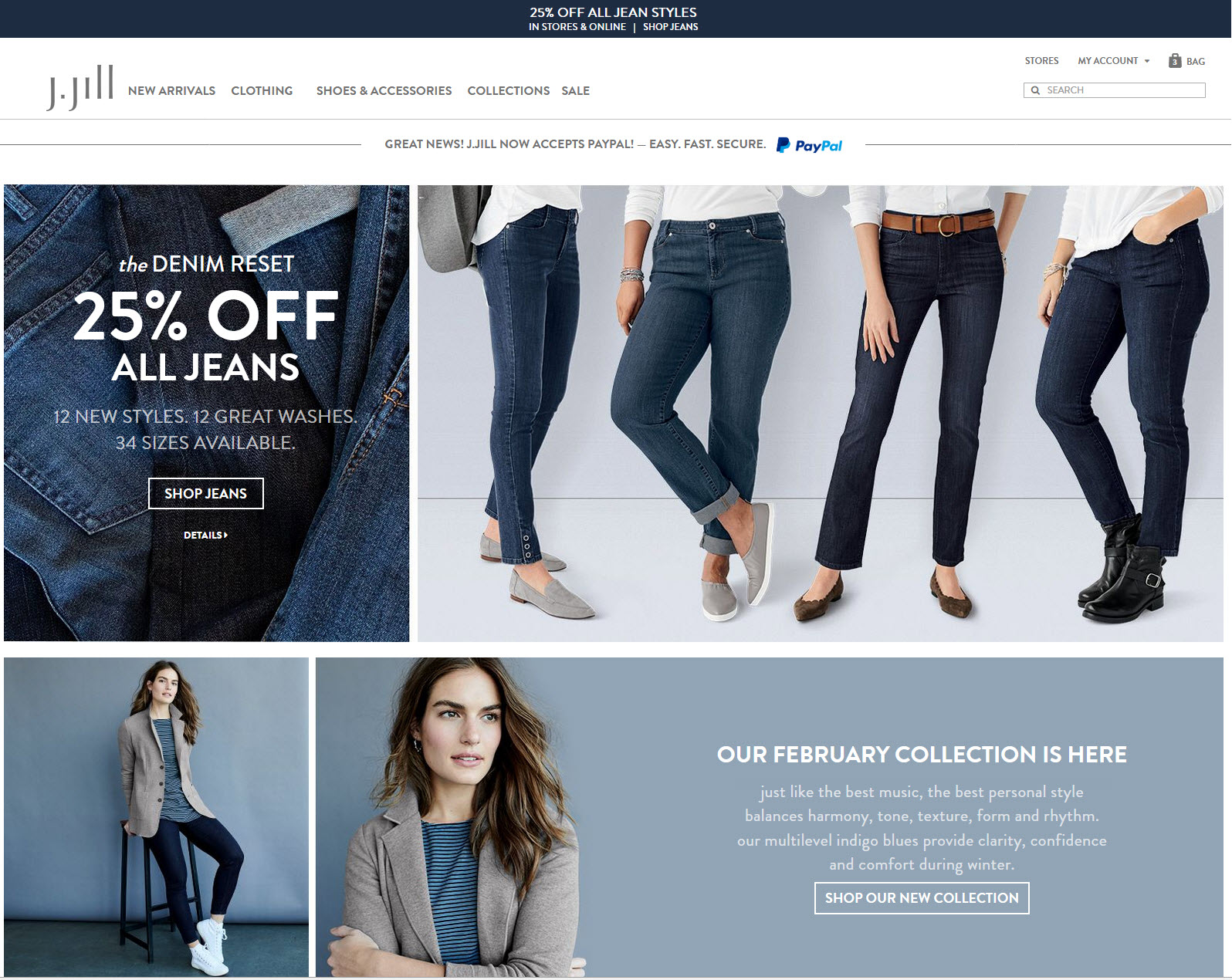The J.Jill webpage opens with a prominent blue banner across the top, announcing a "25% Off All Jeans" promotion available in-store and online, accompanied by a "Shop Jeans" call-to-action. Beneath this, a white bar features navigation options, including "New Arrivals," "Clothing," "Shoes and Accessories," and "Sale." It also includes site search functionality and links to the store's main sections, "My Account," and "Bag."

A horizontal divider follows, and the text "Great News! J. Jill now accepts PayPal - Easy, Fast, Secure" is displayed alongside the PayPal logo. Below this message, a detailed close-up image showcases the back pocket of a pair of jeans with the caption "The Denim Reset: 25% Off All Jeans. 12 New Styles. 12 Great Washes. 34 Sizes Available." Located below this is a black button labeled "Shop Jeans" and an informative link for more details.

Further down, a vibrant image displays four individuals wearing different styles of jeans paired with white shirts and various types of shoes. Below this, an image on the left depicts a woman casually seated on a stool. She is dressed in a pea coat, jeans, and white sneakers. Beside her, a close-up shot captures her face, her jacket, and her crossed arms. Adjacent to this image, text announces "Our February Collection is Here," followed by a white button prompting users to "Shop Our New Collection." This section is set against a blue background.